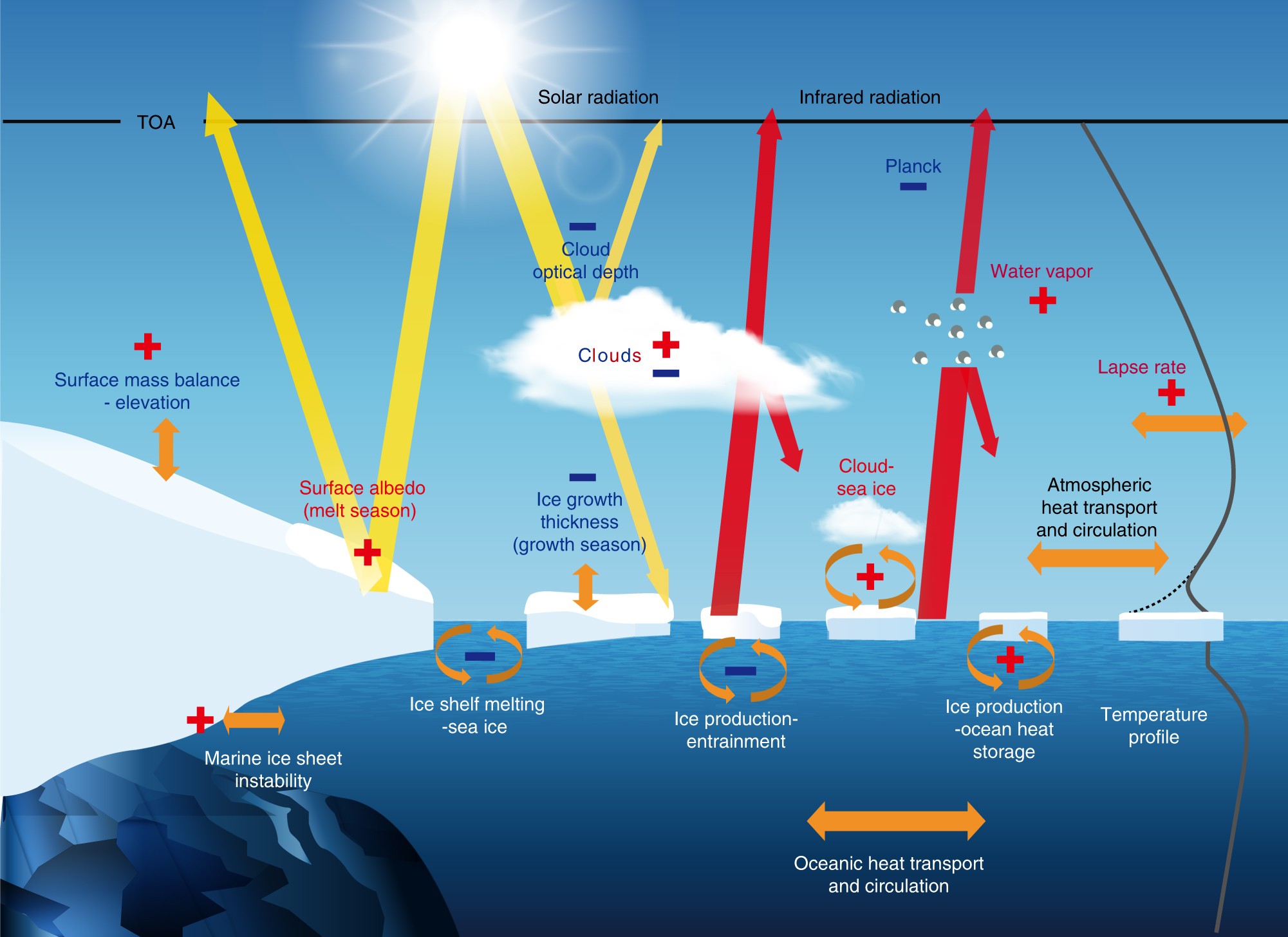This image is a detailed scientific diagram illustrating the heat circulation between solar radiation, ice melt, and oceanic processes. At the center, an iceberg is seen in the ocean, surrounded by smaller icebergs. The scene is labeled with multiple components to explain their interactions. On the top left of the image, some white ice is marked 'surface mass elevation' with a red plus sign on top. The ocean below also contains ice labeled with a yellow line denoting 'ice growth thickness, growth season.'

Above this, the sun radiates solar energy, depicted by a yellow arrow labeled 'solar radiation,' which points downward. A black line beneath the sun, labeled 'T-O-A,' signifies the top of the atmosphere. Red arrows labeled 'infrared radiation' are shown emanating from the iceberg, illustrating heat emission. In the air, clouds and water vapor are present, contributing to atmospheric processes.

At the bottom of the diagram, a large orange double-sided arrow labeled 'ocean heat transport and circulation' runs horizontally, indicating the movement of heat within the ocean. The entire background is a gradient of blue, signifying the ocean and sky, while the diagram's annotations appear in red, yellow, and black for clarity.